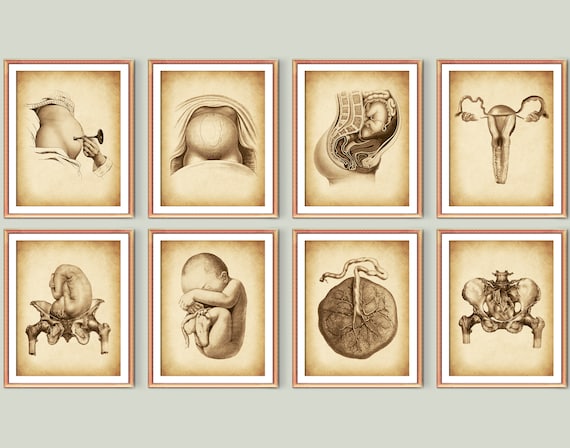The image is an intriguing collage of eight picture frames, each containing detailed anatomical drawings and photographs that collectively depict various stages and elements of the human reproductive cycle. The frames are arranged in a 2x4 grid, four on top and four on the bottom, all encased in light wood with white borders framing each image.

Starting from the top left, there is an old-fashioned photograph of a man holding a stethoscope-like device to a pregnant woman's stomach, suggesting the image's vintage nature. To its right, the next image is a close-up of a pregnant woman's belly. Following that, the third frame contains a side profile diagram of a woman carrying a baby, detailing the baby's position within the womb. The final frame on the top row shows the female reproductive anatomy.

On the bottom left, the first picture is a drawing of a baby resting on top of a pelvic bone. To its right, the next image depicts a baby inside what appears to be a womb, though not explicitly detailed as such. Next in line is an illustration of the placenta, and the bottom right frame shows a skeletal structure highlighting the area where the baby would be carried.

This comprehensive and chronological display provides a fascinating visual representation of the human reproductive process, from conception to pregnancy and anatomy.